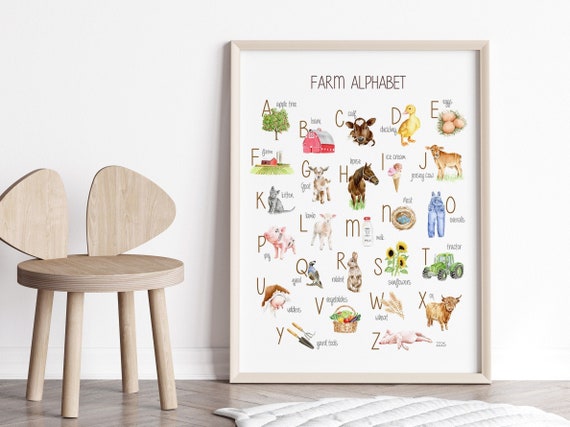In the cozy, minimalist room, a light beige wooden stool with four legs and a unique guitar-pick-shaped backrest stands out on the gray hardwood floor. The stool, likely sized for a toddler, is positioned near a white baseboard and a white wall, which provide a clean backdrop. Nearby, partially visible on the bottom right, is a modeled white rug, adding a touch of warmth to the space.

Dominating the right center of the frame is a tall, vertical rectangle poster, elegantly encased in a light gray wooden frame. This poster features a "Farm Alphabet" title in dark text at the top. Against its black background, brown text labels each of the letters from A to Z, accompanied by charming farm-themed illustrations. The letters are listed in rows, each introducing a whimsical element of farm life: A for apple tree, B for barn, C for cow, D for duckling, and so forth, culminating with Z for ZZZZ, depicted by a sleeping pink pig. The carefully curated details and gentle colors of this setup perfectly complement the serene and playful atmosphere of the room.